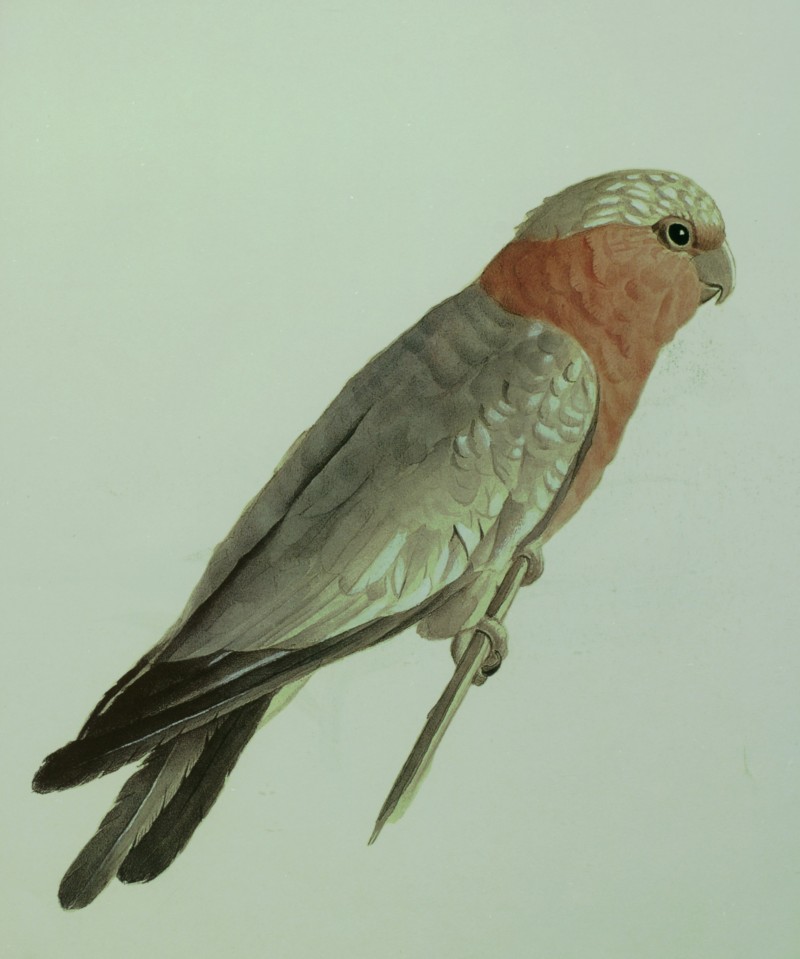The detailed painting depicts a bird perched on a branch, possibly a stick or bamboo shoot. The bird, shown in profile and gazing ahead with a calm and serious demeanor, features a mix of greenish and brownish feathers, with darker hues towards its tail. Its breast and neck exhibit a distinct red or pastel red coloration. The feathers transition from white or beige to dark gray or black towards the wingtips and tail. The bird's small, curved beak and large, prominent black eye are striking against its muted green-toned surroundings. The background is a light blue or gray, enhancing the solitary and serene atmosphere of the image.